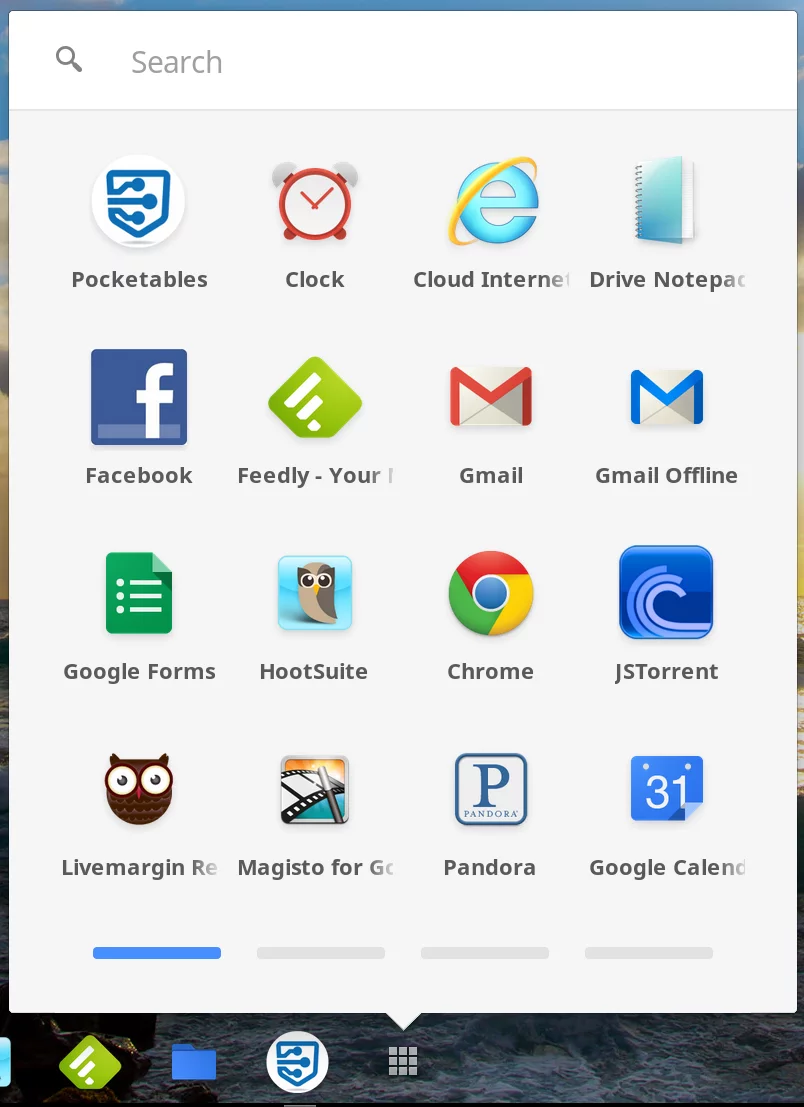This image is a screenshot from an Android tablet's home screen, cropped in a way that only a small portion of the edges is visible. The primary focus of the image is the opened app drawer, which has a white background. This drawer has been accessed by tapping an icon resembling a cube with a tic-tac-toe layout, typically found at the bottom of the screen.

In the app drawer, we are on the first page of four total pages, indicated by four dots at the bottom, with the first dot highlighted in blue. The visible apps on this page include a mix of Google-related applications such as Gmail, Gmail Offline, Google Chrome, Google Calendar, Google Forms, and others like Facebook, Cloud Internet, Drive, Notepad, Pocketables, Live Margin, Pandora, and JS Torrent. 

Given the combination of Android and Google-related apps along with the layout and interface, this screenshot likely originates from an Android tablet or possibly a Chromebook in tablet mode.